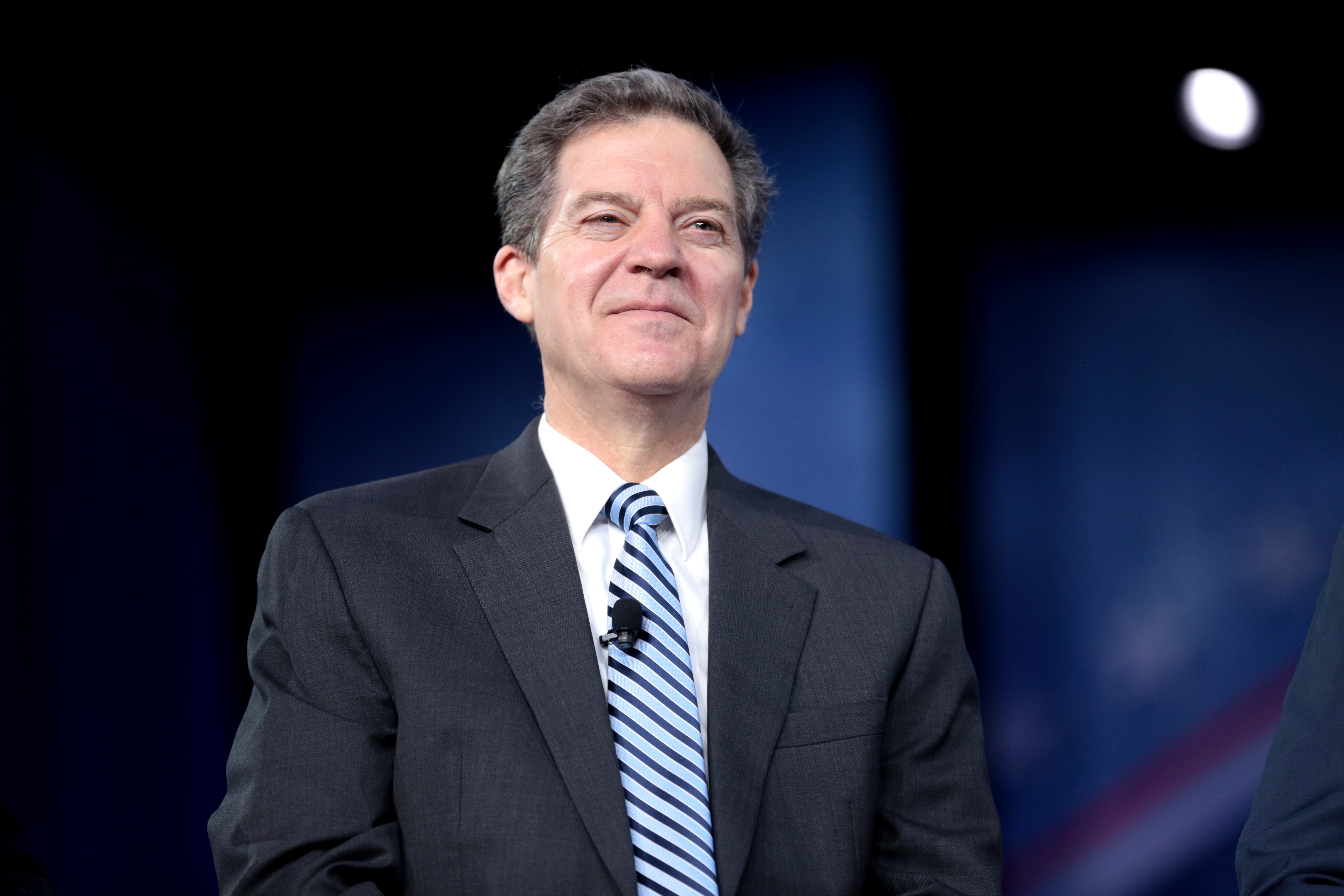In this dimly lit photograph, various tones of dark blue and black create a somber background, punctuated by lighter shades of blue. A small, bright speck in the top right corner likely represents a distant light source. The centerpiece of the image is an elderly man with a mix of dark grey and light grey hair. His gentle, soft smile conveys warmth as he looks directly at the camera. He is dressed formally in a crisp white collared shirt paired with a dapper tie featuring alternating dark blue and light blue stripes. Over his shirt, he wears a polished black business jacket. A microphone is clipped to his tie, suggesting he may be speaking or preparing to address an audience.